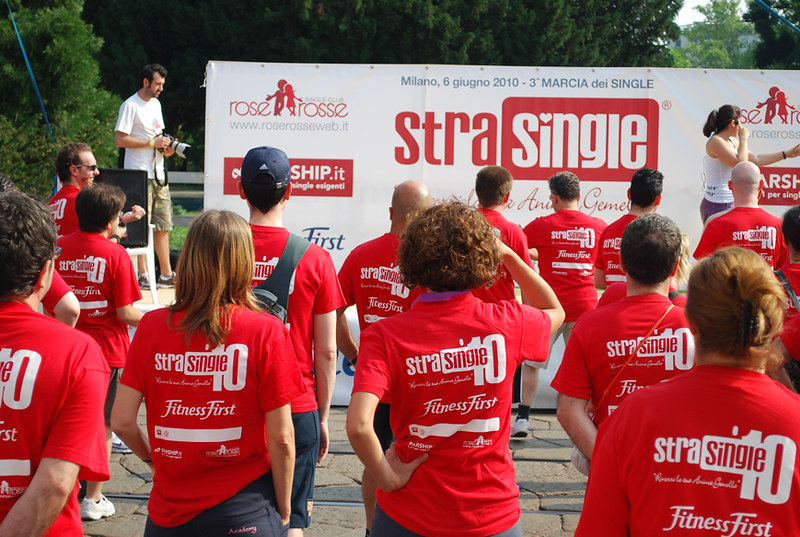This full-color landscape photograph captures an outdoor event centered around fitness, featuring a stage and a large white banner with prominent red text and logos that read, “Straw Single 10 Fitness First” and other inscriptions such as “Milano 6” and “2010 3 Marcia Day Single.” The image is taken from behind the crowd, revealing the backs of numerous attendees, both men and women, all clad in red t-shirts with white text matching the banner's message. To the left of the stage, a man in a white shirt and camo pants is holding a large camera, while to the right, a woman with a headset, presumably directing the event, gazes off to the side. The stage backdrop features foliage and trees, enhancing the outdoor setting. The crowd is a mix of people with various hairstyles and accessories, all seemingly focused on the stage, highlighting the engaging nature of this organized fitness activity.